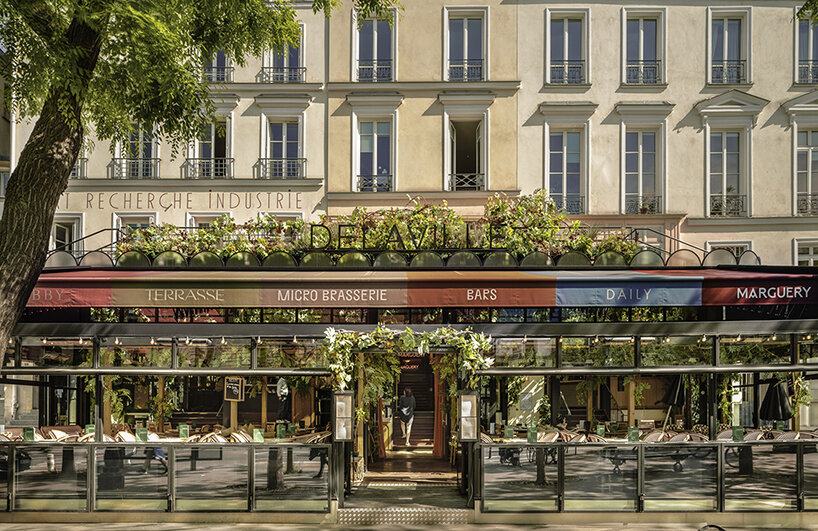The image depicts a lively city sidewalk on a sunny day, likely in a French-speaking area, showcasing the charming architectural and cultural elements typical of such locales. The street is lined with a series of quaint storefronts, each with its unique signage; names like Delaville, Taurasi, Micro Brasserie, Bars, Daily, and Marguerite can be seen prominently displayed, inviting patrons to explore the various offerings. Above the storefronts, the building facade is painted in a soothing light peach color, adorned with two to three rows of large windows and a couple of balconies, all arranged horizontally across the structure. These architectural details add to the picturesque charm of the scene. 

In front of the shops, outdoor café seating areas spill onto the sidewalk, creating an inviting atmosphere for passersby to sit and enjoy the day. A woman stands at the center of the image, heading towards one of the storefronts, stepping up a couple of stairs and through a doorway. Her presence adds a human element to the busy scene, emphasizing the area's bustling nature. To the left of the image, a tree provides some greenery, complementing the plants and foliage scattered throughout the scene, both in front of and above the storefronts, contributing to the overall lively and fresh atmosphere of this beautiful day in the city.